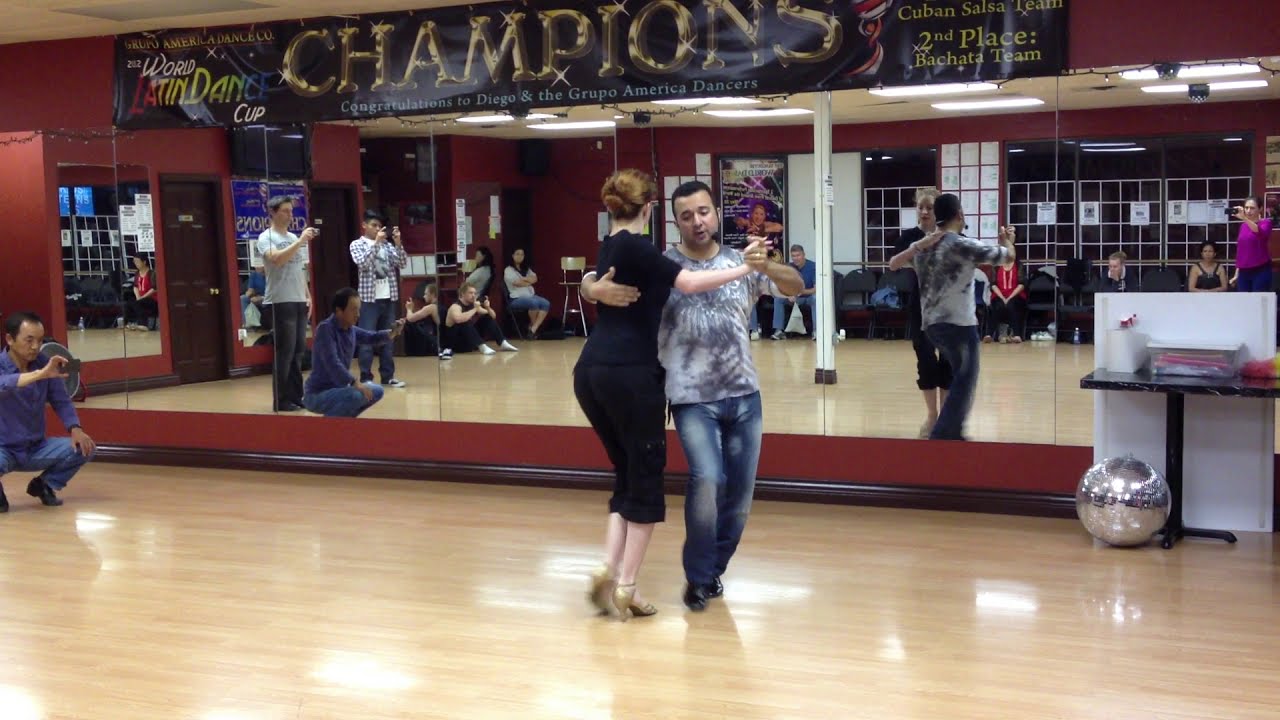In the photograph, a couple is captured mid-dance in a bustling dance studio where several onlookers are either seated on the floor or in chairs, engrossed in their performance. The man, wearing a blue and gray tie-dyed t-shirt, faded Levi’s jeans, and black dance shoes, is identifiable by his headset microphone as he holds his partner. The woman, elegant in a black dress that slightly extends past her knees and paired with tan shoes, faces a mirrored wall adorned with a prominent banner. The banner applauds the "World Latin Dance Cup champions" with a congratulatory message to "Diego and the Grupo America dancers." The room's vibrant energy is emphasized by a man kneeling in the left corner recording the dancers, and the reflection in the mirror showing others also engrossed in capturing the moment. A table on the right holds a disco ball, adding to the celebratory atmosphere with its silver glint. The scene is a vivid blend of colors like blue, beige, reddish-brown, silver, gray, white, black, gold, red, and purple, contributing to an atmosphere of festive anticipation and lively engagement in this indoor dance hall.